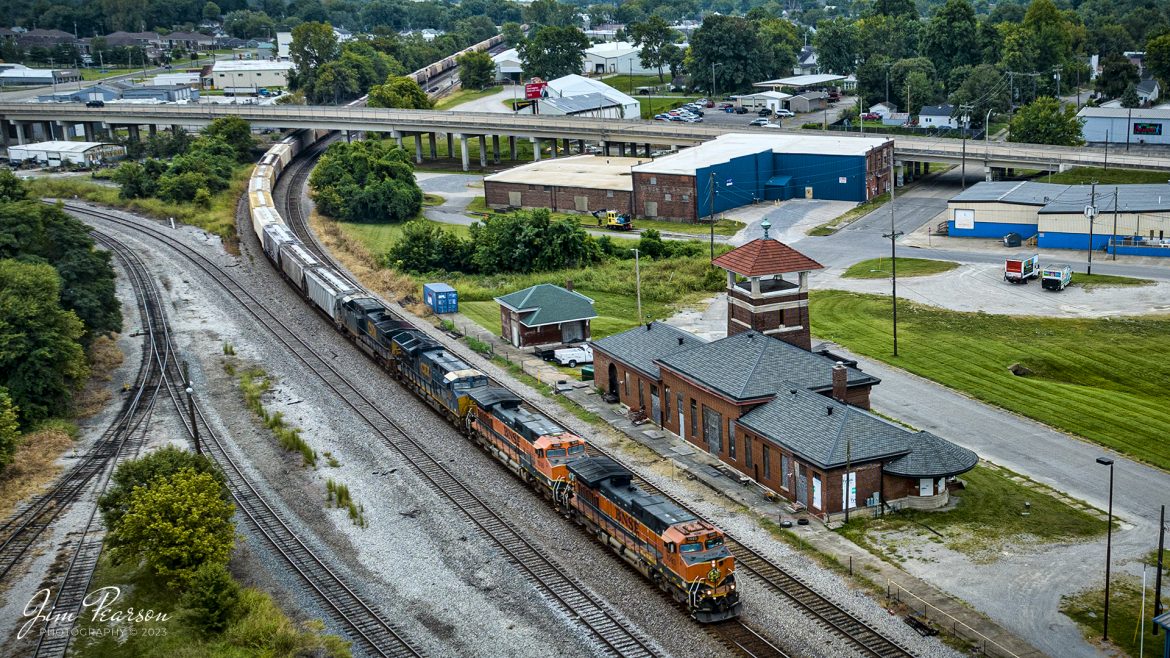This detailed aerial photograph captures a vibrant scene in a suburban town, emphasizing the central feature of an active railway line running through the middle of the image. A prominently visible train with orange and black compartments traverses the tracks. The scene includes a notable brown, red-brick building with a gray rooftop and a red watchtower, possibly indicating a significant structure like a train station. Surrounding this building are various other structures, including houses with green roofs and buildings that appear to be manufacturing facilities or warehouses, one of which has blue walls. Further details reveal a freeway running parallel to the tracks, interspersed with passing cars. On the left side of the image, abundant trees and greenery are visible, adding to the overall suburban feel. The lower left-hand corner prominently features the white text "Jim Pearson Photography, 2023," identifying the photographer and the year the photograph was taken. The elevated perspective, possibly from a drone, provides a comprehensive and dynamic view of the railway system amidst the town's infrastructure during daytime.